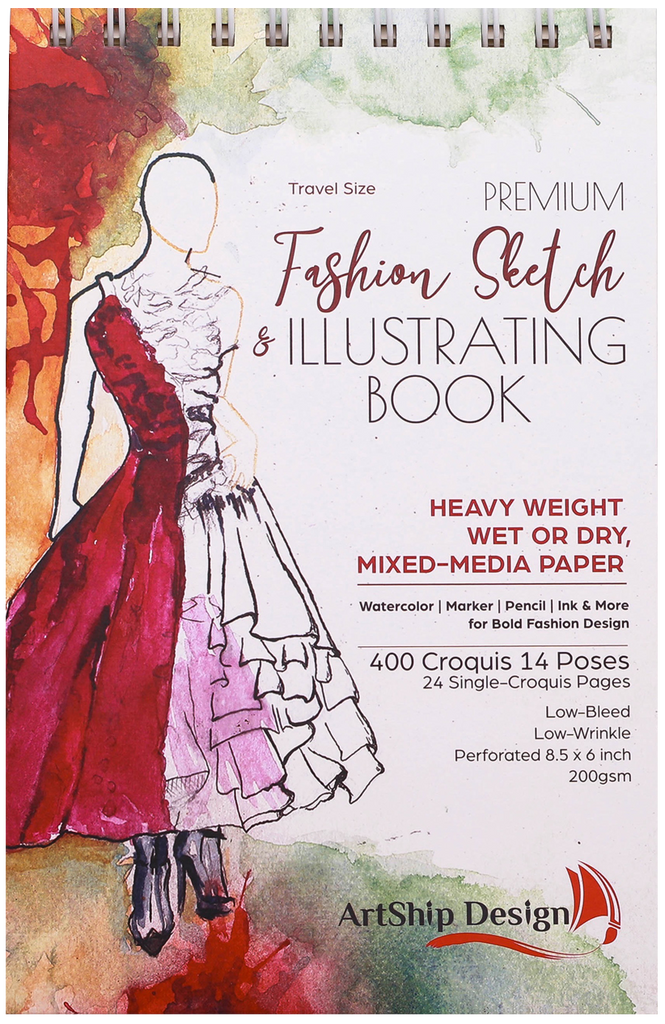The cover of this 8.5 x 6 inch sketchbook from Art Ship Design features an artistic, partially watercolor, partially sketched illustration of a dress, depicted on either a person or mannequin. The dress is primarily red and white with an artistic, painted appearance, accompanied by a few additional colors like orange and green. The sketchbook is travel-size and premium, specifically titled "Fashion Sketch and Illustrating Book." It boasts heavyweight, wet or dry mixed-media paper suitable for watercolor, marker, pencil, ink, and more, ensuring low bleed and low wrinkle. The cover also details the inclusion of 24 single pages featuring 14 different poses. The top edge reveals rings, suggesting a binder-style design for easy use.